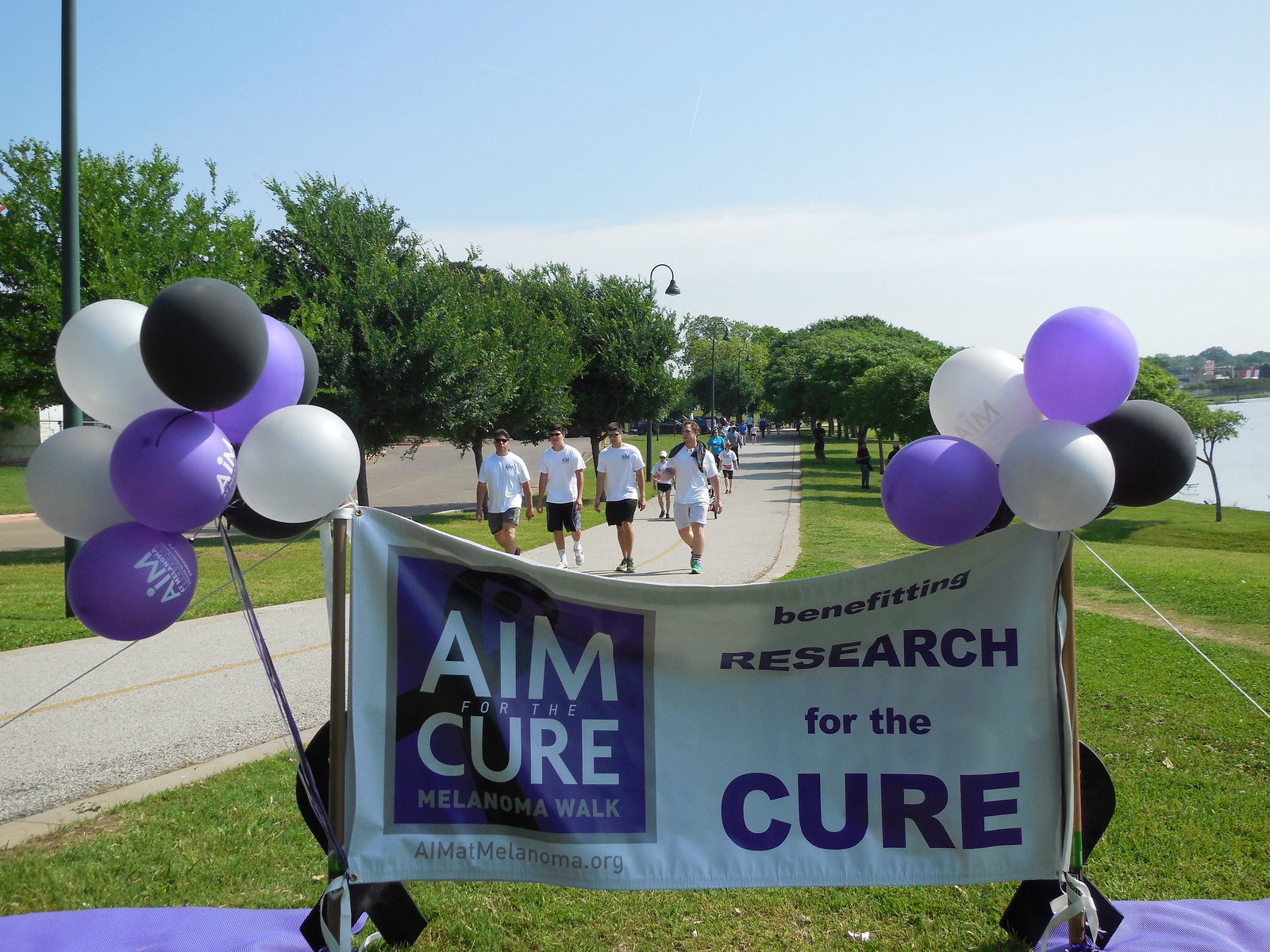The image portrays a vibrant scene at a park, where a large white banner heralds the "Aim for the Cure Melanoma Walk." The banner, mounted between two poles adorned with clusters of purple, black, and white balloons, features a prominent purple square and text that reads "Aim for the Cure Melanoma Walk," along with the website "aimatmelanoma.org" and the phrase "Benefiting Research for the Cure." The event aims to raise funds for melanoma research, bringing together a community united in their determination to find a cure for this rare disease. 

In the background, the park's green landscape comes to life with a walkway running down the center, flanked by lush green grass and mature trees stretching all the way to a serene lake. The sky above is a clear blue with a few white clouds, suggesting a pleasant day. Numerous participants, all donning white t-shirts and an assortment of white or black shorts, stroll along the path. Street lamps and a curving lamppost add a charming touch to the scene. The atmosphere is lively and filled with purpose, as the walkers, bound by a shared mission, advance towards the goal of eradicating melanoma.